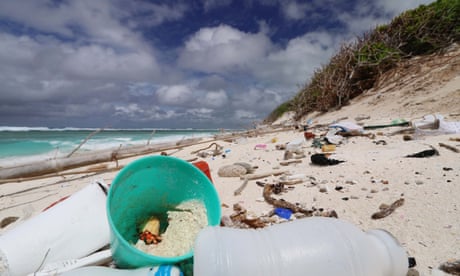This photograph captures a desolate beach strewn with various forms of debris and discarded objects. In the foreground, a green bucket filled with sand, likely used for building sandcastles, stands out among the litter. Prominent amidst the rubbish are a white plastic water bottle, cups, and other waste, contributing to the beach's cluttered appearance. The sand is light-colored but marred by sticks, driftwood, and colorful trash, including hints of pink, black, yellow, and blue objects scattered throughout. The ocean, a striking aqua color, stretches out to meet a dark blue sky filled with white clouds. Above the beach, a grassy cliff frames the scene. Despite its picturesque natural elements, the overall beauty of the beach is significantly diminished by the visible pollution.